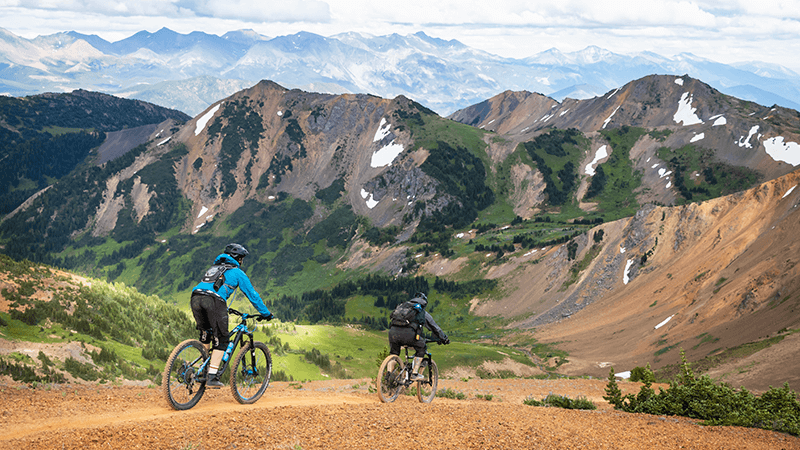This photograph captures two mountain bikers navigating a red clay path in the countryside. The rider in front is wearing a gray shirt, black pants, a helmet, and has a backpack, while the rider in the back sports a turquoise long-sleeve shirt, black knee-length shorts, a helmet, and a backpack. The path they are biking on is surrounded by grassy shrubs on the lower right corner, leading to grassy covered hills on the left, which ascend towards dark gray, snow-capped mountains. The background showcases additional mountains with a mix of grayish-brown and white snowy peaks, enveloped in silvery blue clouds. The captivating scene is accentuated by the open sky visible in the far distance.